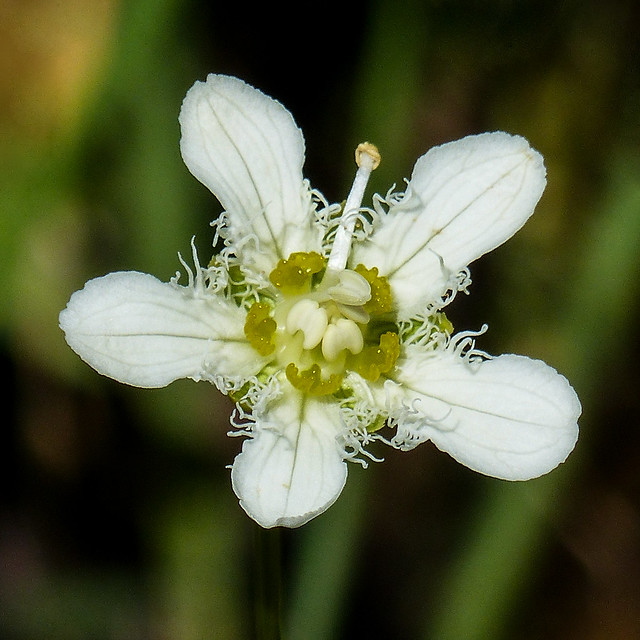This close-up image showcases a unique and intricate white flower, adorned with five pointed petals arranged in a star-like formation. Each of the petals, which appear almost fabric-like, are spaced at intervals resembling a clock face: 11 o'clock, 2 o'clock, 4 o'clock, between 6 and 7 o'clock, and 9 o'clock. They gently bow outwards towards the ends. Tiny, curled white strands, resembling ribbons or confetti, sprout from about halfway up each petal, adding to the flower's detailed texture.

The flower's center is a striking composition of color and structure. Embedded within are three small, nascent white petals, surrounded by translucent green, jelly-like growths that emit a yellowish-green hue. Rising from this central area is a slightly bent, white column topped with a yellow tip. This arrangement of delicate elements makes the flower's core appear both protected and intricate.

Set against a dark, blurred background of green and black with a touch of brown in the left-hand corner, the flower stands out brilliantly, utilizing a bokeh effect that emphasizes its delicate beauty and fine details.